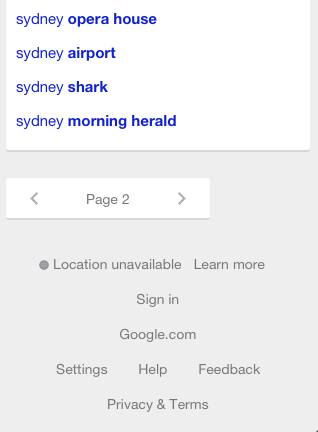In this image, it appears a search interface is displayed without a visible search bar, showing a list of four distinct options, each presented as names. The options listed are:

1. **Sydney Opera House** - where "Opera House" is highlighted in bold and blue text.
2. **Sydney Airport** - "Airport" is bold.
3. **Sydney Shark** - "Shark" is emphasized in bold.
4. **Sydney Morning Herald** - with "Morning Herald" bolded and colored blue.

Below these options is a navigational element labeled "Page 2," flanked by arrows for navigating left and right. There is also a message indicating "Location unavailable" with a "Learn more" link beside it. Centrally positioned below this message is a "Sign In" button, and beneath that, the URL "google.com" is displayed prominently. At the bottom, options for "Settings," "Help and Feedback," and "Privacy and Terms" are aligned centrally.

The backdrop of the image is predominantly gray, except for the white background which highlights the listed search results and the "Page 2" section. This image seems to be a cropped screenshot where the upper part containing the search input field is missing, leaving only the search results visible. The cutting-off of the top part suggests the image was intentionally modified to focus solely on the search results.